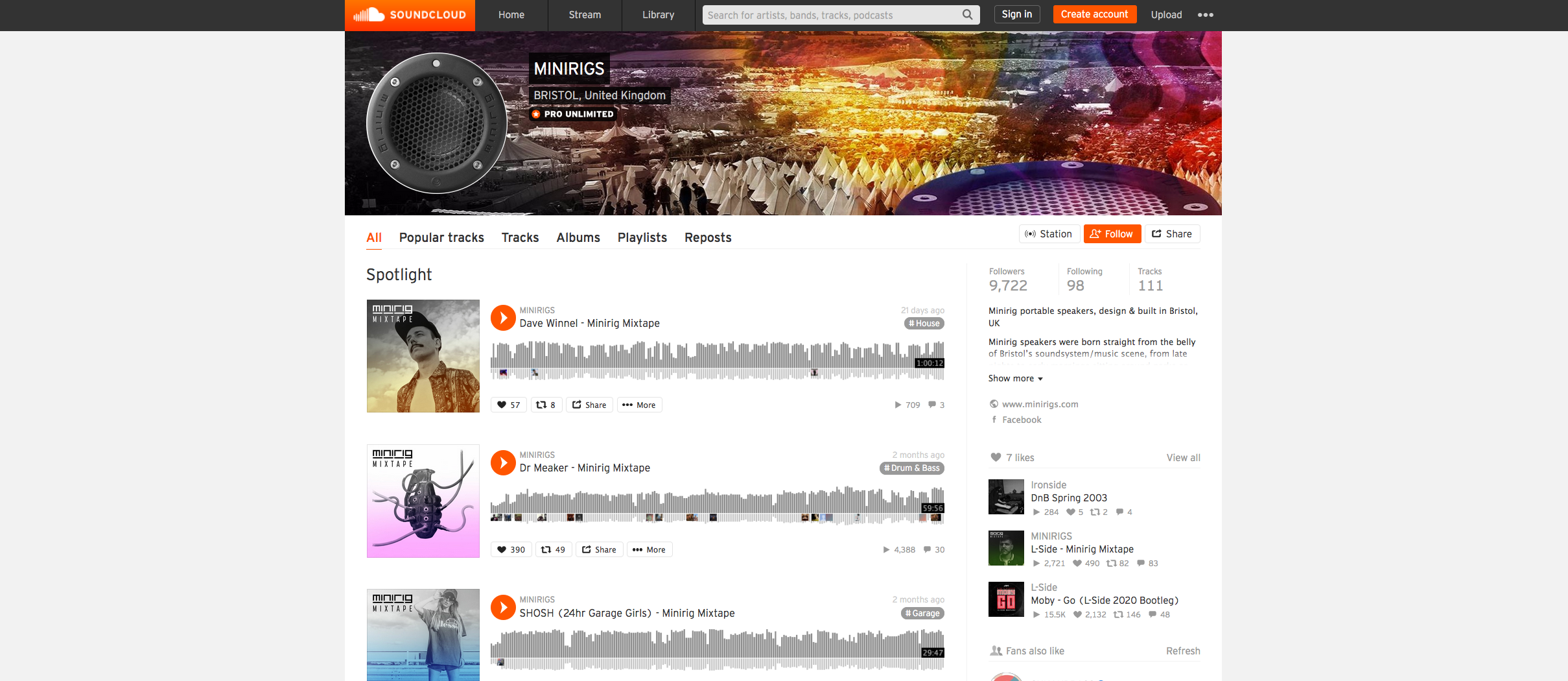The image depicts a SoundCloud webpage, a platform dedicated to musical artists and creators. Dominating the header is the SoundCloud logo set against an orange background. Accompanying this are various navigational tabs and a search bar for exploring the site. 

Directly below, there is a visually striking, ambient image characterized by rainbow-like swirls and abstract mountain shapes, giving it an AI-generated, ethereal feel. On the left side of this image is an icon resembling a speaker labeled "Minirigs," indicating the artist or speaker from Bristol, United Kingdom.

Further down, a row of tabs is displayed, offering quick access to "All," "Popular Tracks," "Tracks," "Albums," "Playlists," and "Reposts," organizing the content methodically. Below these tabs, three audio tracks are listed, each accompanied by distinct images: one features a portrait of a man, another depicts a grenade, and the third displays a mysterious figure.

To the right of these tracks, there are metrics showing the engagement for this page, such as counts of plays, likes, and potentially other audio files. However, these details are small and difficult to discern.